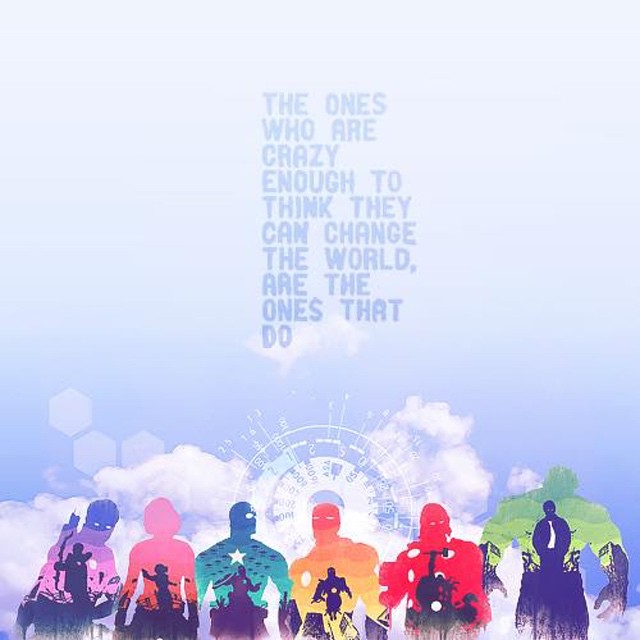The digital image is a vertical, rectangular illustration exuding a motivational aura. The background is a gradient of various shades of light blue, giving it a slightly cartoonish feel, and it features a sky-like backdrop. Toward the bottom half, a layer of clouds or perhaps smoky mist adds a dreamy, ethereal touch. The inspiring quote, "The ones who are crazy enough to think they can change the world are the ones who do," is prominently displayed in darker blue, horizontal rows from the top to the center of the image. At the bottom, seven figures stand out. These figures are vibrant silhouettes in a spectrum of colors including light purple, pink, turquoise, orange, red, dark blue, and green, with additional hues like gold within their outlines. Some figures possess superhero-like characteristics, with inner representations of themselves on their chests. These outlines give the impression of action figures or superheroes, enhancing the image's powerful and encouraging theme.